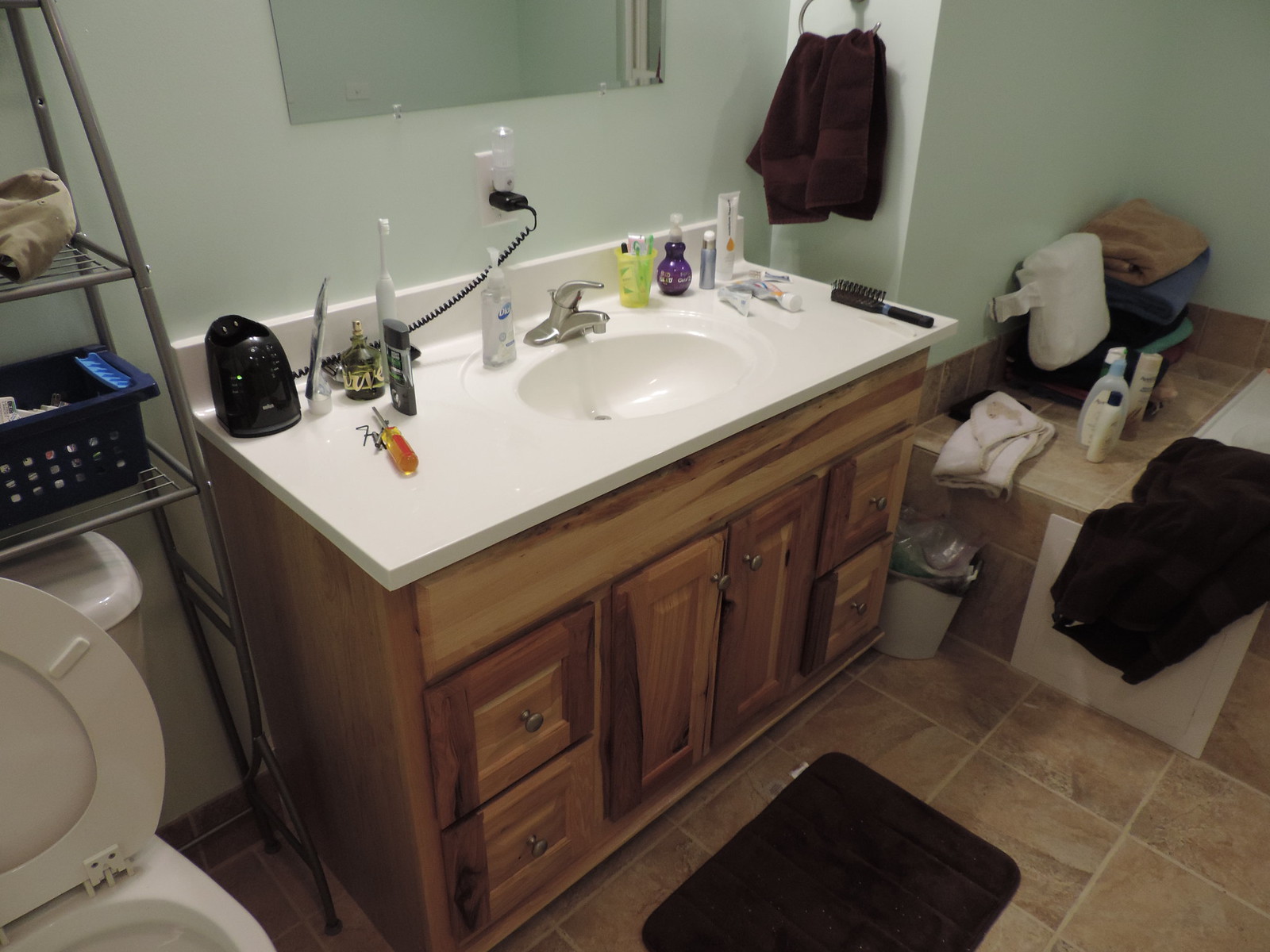An indoor color photograph captures a detailed perspective of a bathroom, focusing primarily on the sink and its surrounding cabinet. Taken from a 45-degree angle, the image provides a comprehensive view from the front-left side of the bathroom.

In the lower-left corner, a portion of the toilet is visible, with the toilet seat in an upright position. Behind the toilet, a gray wire rack with two shelves stands against the wall. On the bottom shelf sits a black plastic container, while the top shelf holds what appears to be a sock or a similar item.

On the countertop, various items are spread from the foreground to the background. The closest item is a charger, likely for an electric shaver or toothbrush. Next to it stands a nearly empty toothpaste tube, balancing on its cap. A screwdriver, handle facing the photographer, rests with several screws nearby. A stick of deodorant, encased in gray, stands beside an electric toothbrush, which is white in color.

Near the sink, a clear bottle of Dial hand soap is positioned conveniently. The sink itself features a silver faucet with a single handle. To the right of the faucet, a cup holds several toothbrushes. Further right, there is a purple bottle—potentially of hand sanitizer or cleaner. Additionally, two small bottles are aligned beside it, with a brush sitting at the far right corner of the countertop.

The pale green wall above the sink includes a mounted mirror, reflecting parts of the bathroom. In the image's right corner, the tiling of a bathtub area is noticeable, with neatly folded towels placed on the tile edge. In the foreground, near the right side, a mat lies in front of the cabinet on square brown tiles, completing the floor's appearance.